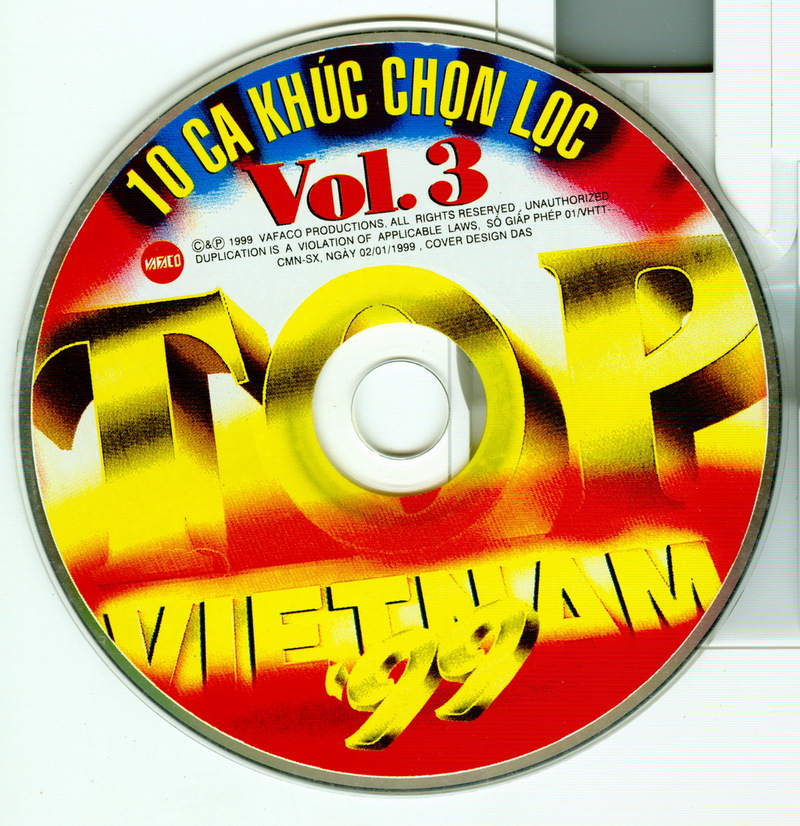The image depicts a compact disc (CD) with a predominantly white and gray background, possibly resting on a white device or table. The CD boasts a mix of vibrant colors, including bright yellow, red, blue, white, and black, with yellow being most prominent at the top. The CD is designed with a silver bezel surrounding it. 

At the top of the CD, in large red letters, it reads "Tên Ca Khúc Chọn Lọc," followed by "Volume 3." Midway across the CD in gold letters, it says "TOP," and below that, "Vietnam 99" is inscribed against a red background. Additional fine print on the CD includes the text "1999, Vafaco Productions, All rights reserved. Unauthorized duplication is a violation of applicable laws," along with "02-01-1999" and "Cover design by DOS." This indicates that the CD is a compilation of top Vietnamese songs from the year 1999, produced by Vafaco Productions.